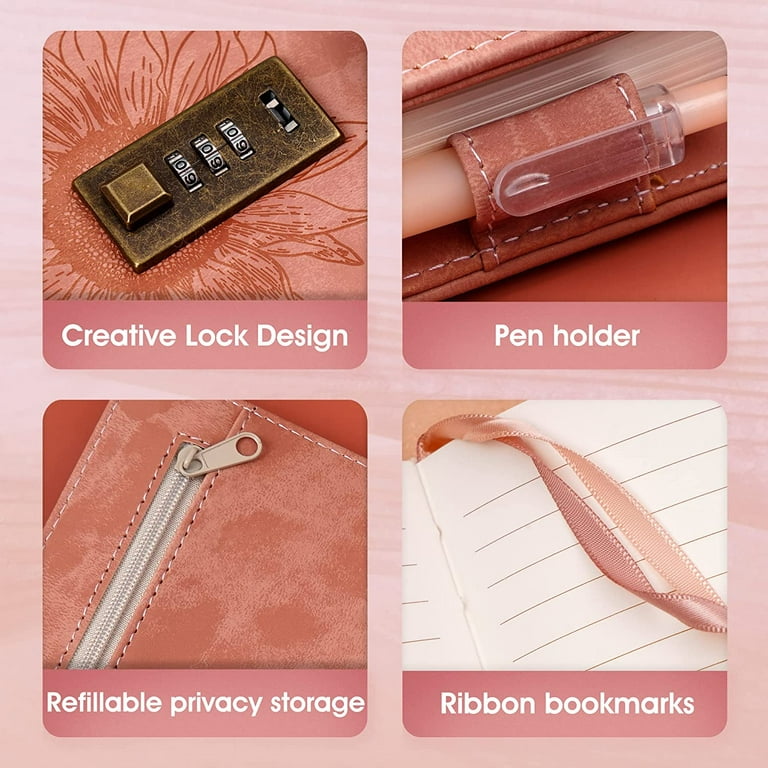The image showcases four distinct product photos of a notebook or diary, arranged on a single square background adorned with pink and white stripes. Each photo is square with rounded corners and highlights a unique feature of the product. Starting from the upper left and moving clockwise, the features are: 

1. A creative lock design illustrated by an image of a combination lock.
2. A pen holder, displaying a pen secured within a leather loop.
3. Ribbon bookmarks, shown in the bottom right corner to indicate their functionality.
4. A refillable privacy storage compartment, featuring a zippered pocket for secure storage.